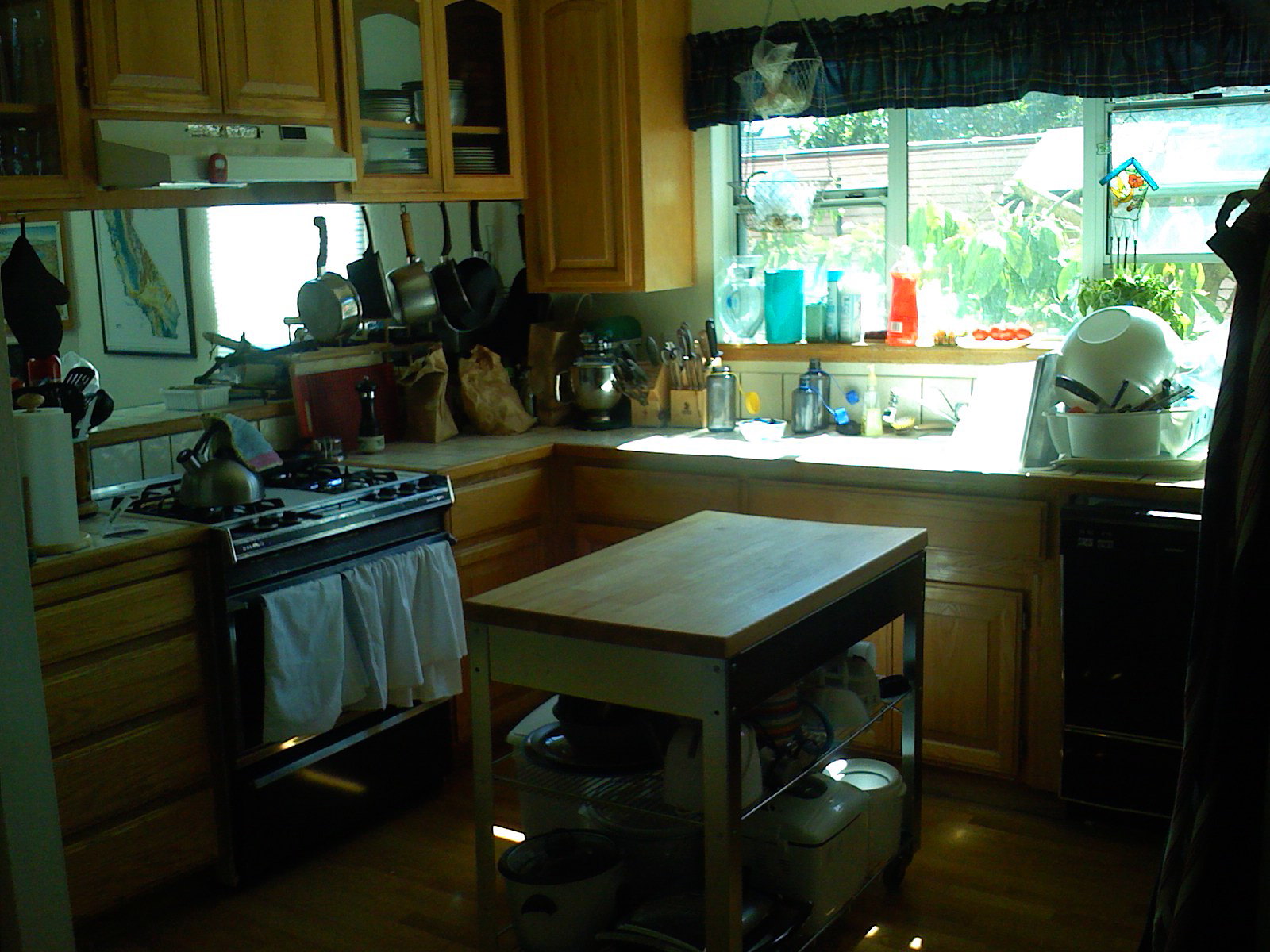This image depicts a bustling and well-used kitchen, bathed in natural daylight streaming through large windows. The light casts an intricate interplay of shadows across the room. Central to the kitchen is an island table with slatted shelves underneath, filled with assorted ceramic cookware. The space is lined with numerous wooden cupboards and drawers, meticulously arranged yet giving a sense of organized chaos. Pots and pans hang above the countertops, alongside an array of cutlery and knives. Canvas cloths hang near the oven, their textures vividly captured in the photograph. Beyond the kitchen windows, a lush garden brimming with greenery and a shed, possibly a greenhouse, can be seen, adding a touch of nature's tranquility to the busy interior.